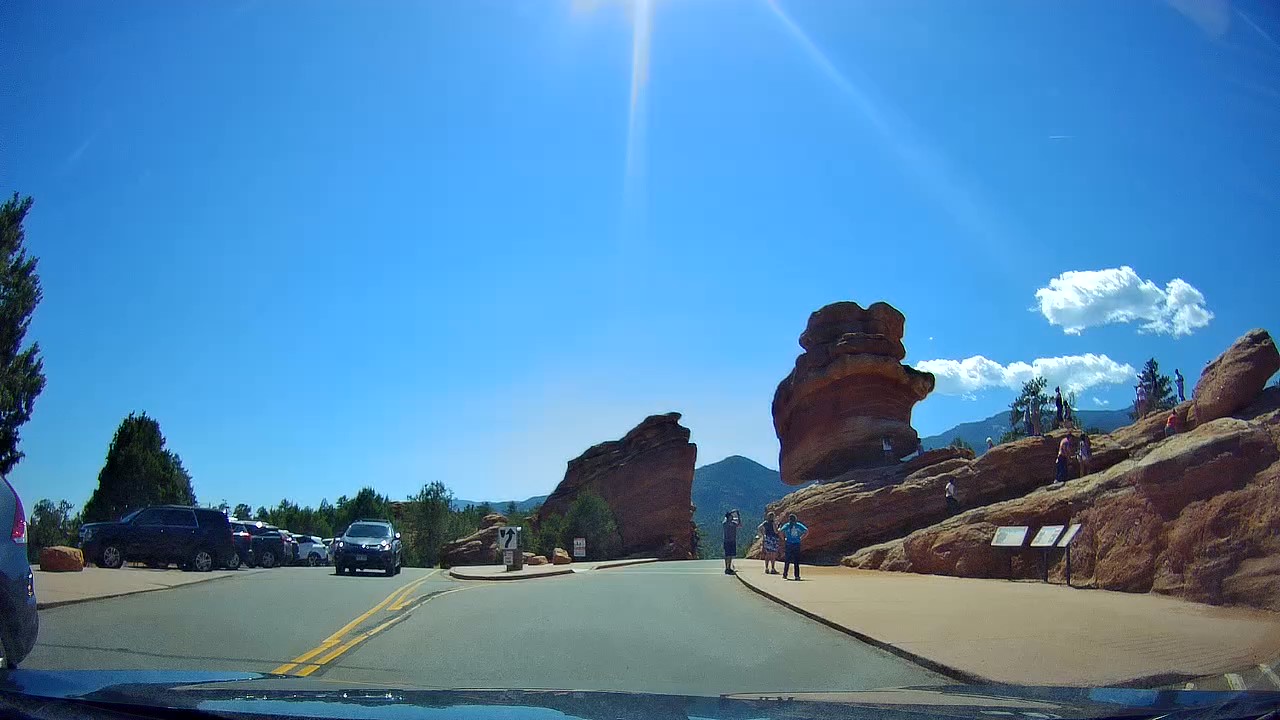A vibrant color photograph taken from inside a vehicle, showing the scenic view of a nature park through the car's windshield. The sun shines brightly in a clear blue sky dotted with a few white clouds. Rocky hills dominate the landscape, with yellow-orange rock formations on both sides. A paved area to the right features a tall stone structure, beside which people are climbing a steep, rocky hill, and others are taking photographs. In the foreground, windshield wipers are visible at the bottom of the image. A road curves through the center of the image, flanked by numerous parked cars, trees, and three small podiums with signage. To the left, another road, lined with more cars and trees, leads towards majestic mountains in the background. The scene is lively with individuals capturing the picturesque surroundings while sunbeams stream down, enhancing the beauty of the natural setting.